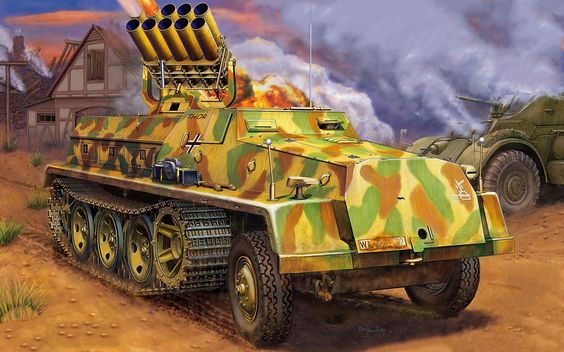This detailed digital artwork depicts a dynamic war scene set in a computer game. The wide rectangular canvas, approximately three inches tall and five inches wide, highlights a camouflaged military tank driving towards the bottom right corner. The vehicle, painted in shades of light yellowish-brown with green and brown spots for a camouflage effect, features two regular rubber wheels with golden rims at the front and at least five wheels at the back, encapsulated by a large black chain.

Patches of green and yellow grass are scattered across the dark lightish brown ground on the left side. The tank's top bristles with weaponry, including a missile launcher array housing ten rockets arranged in two rows of five, one of which is actively launching. Additionally, several cylinder-shaped objects emit vivid bursts of fire. A small viewing turret at the front reveals the face of a driver, peering through a narrow slit.

Prominent text in black reads "Thor" on the left side of the tank, accompanied by a black and white cross with a white outline below it. In the background, to the left, lie the ruins of a house, while to the upper right, obscured by gray smoke and flames, another green tank emerges. The sky in the backdrop transitions through blue and orange hues, intensifying the scene’s dramatic atmosphere.